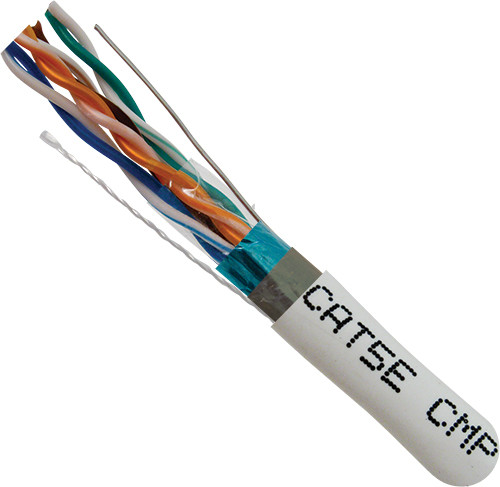The image depicts an Ethernet cable emerging from a white sheath angled from the lower right-hand corner towards the center of the image. The sheath is labeled with the text "CAT5E CMP" in black. Extending from the sheath are twisted pairs of wires in various colors: orange, blue, white, green, and teal. Among these, there is also a solid metallic wire situated to the right. The background of the image is plain white, highlighting the distinct colors and textures of the wires.